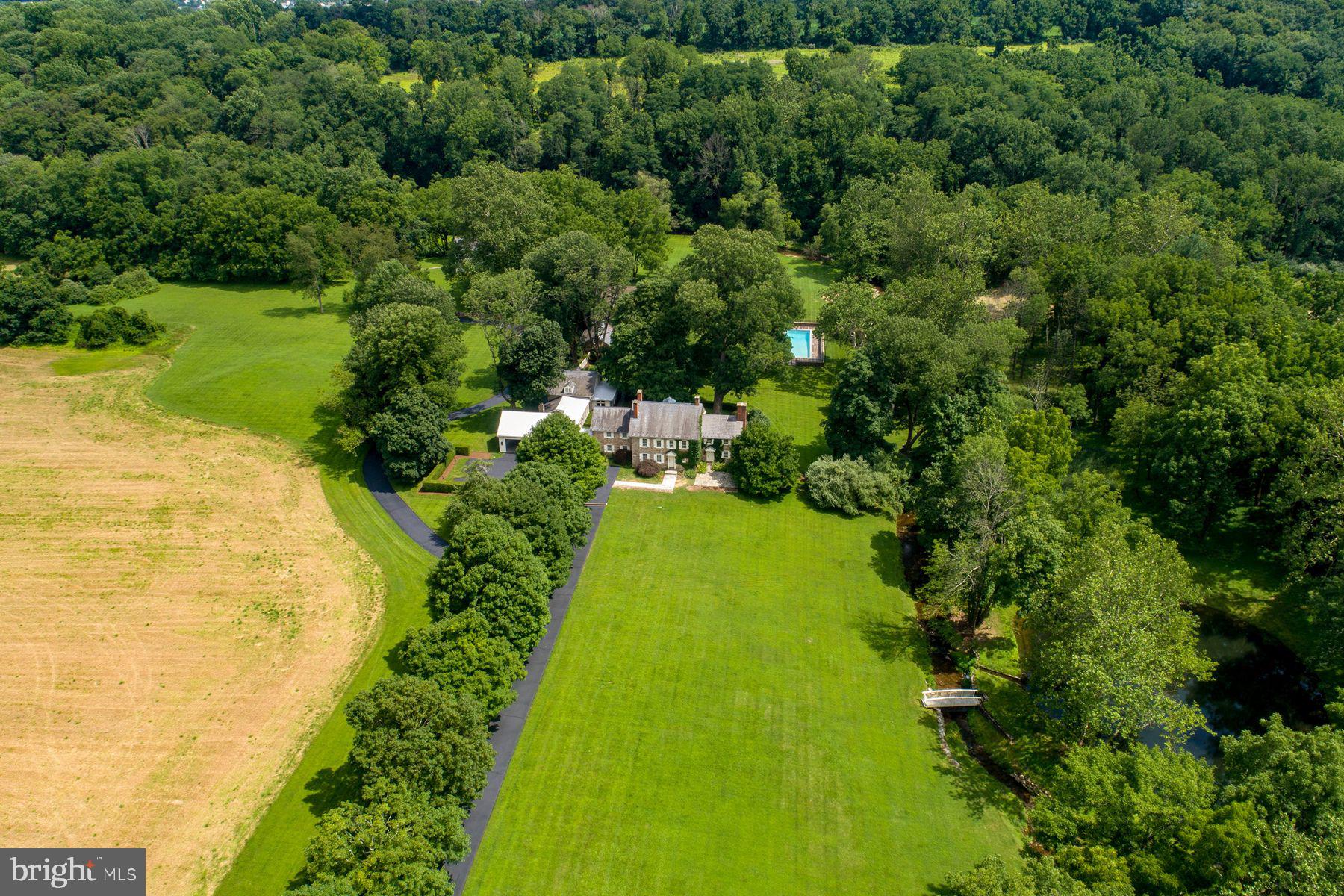This aerial photo, sourced from Bright MLS, showcases a large, meticulously maintained estate surrounded by a dense forest and expansive green lawn. Central to the image is a wide mansion with a distinctive main building, featuring ivy-clad walls on the right side and four chimneys—two on the left side of the main section, one at the top right, and another on the far end of a right-side extension.

Flanking the left side of the mansion is a garage with a white roof, adjacent to which is a guest house. A crystalline pool is visible in the backyard. A long, curved driveway starts from the bottom left of the image, extending to the garage and branching off to circle the property, accentuated by a small concrete path leading directly to the front entrance. 

The property is rich with foliage, large trees lining the left side of the driveway, and a stream running down the right side, crossed by a quaint white footbridge. The estate is bordered by large agricultural fields to the left, contrasting the lush, freshly cut and verdant grass encircling the manor. The setting exudes careful upkeep, tranquility, and natural beauty.